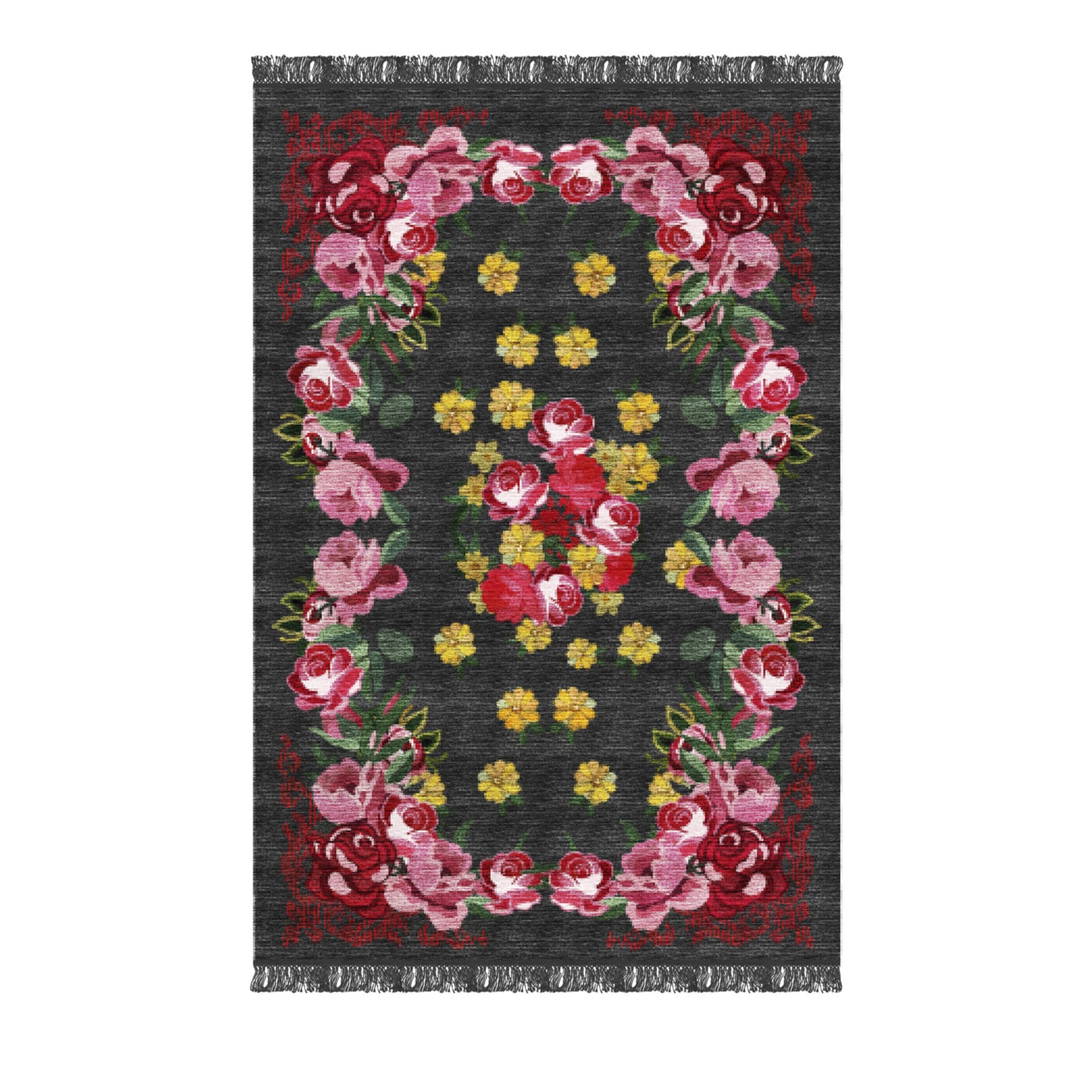This photograph features a detailed, rectangular tapestry that appears to be an area rug or a decorative blanket. The primary background color is a dark gray that extends to form fringed tassels at both the top and bottom edges. A symmetrical floral design frames the piece, creating an outer border of pink roses interspersed with green leaves along the longer sides. Each of the corners is adorned with a striking red rose. The central section of the tapestry showcases a vibrant arrangement of yellow flowers with broad petals, surrounded by clusters of red and pink flowers. The overall design includes hints of dark red along the upper and lower edges, adding depth and contrast to the piece. This detailed and colorful depiction resembles a high-quality stock photo often used for decorative items in living rooms or bedrooms.